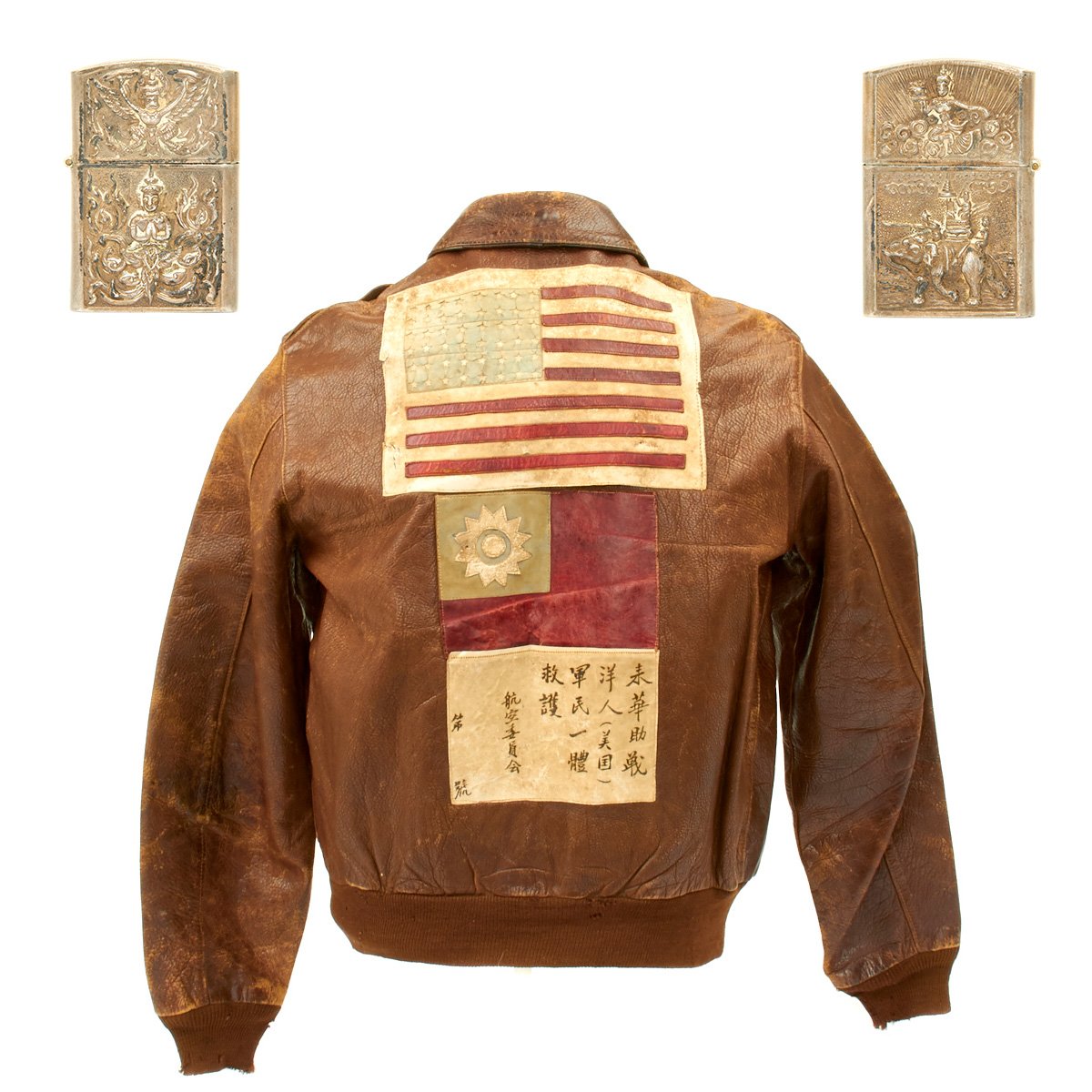This detailed color photograph showcases the back view of an old, medium brown leather jacket, positioned centrally against a plain white background. The jacket itself features a folded over collar, sleeves extending down the left and right sides, and a brown stretchy material at the wrists and waist, some of which is frayed. Prominently displayed across the shoulders is a large, faded, and stained American flag. The flag's red and white stripes contain illegible text, and the traditional blue star field has been replaced with a grey panel that also displays some form of foreign text. Directly underneath the American flag is a rectangular image with a dark red background, featuring a green square in the top left corner. This green square hosts a detailed depiction of a white sun with significant rays. Further down, there is another rectangular panel colored in a whitish cream tint, adorned with horizontal rows of black Asian characters, which are not decipherable. Additionally, on the top left and right corners of the jacket, there are two vertical silver-toned symbols resembling cigarette lighter cases, detailed with brass highlights and etched images of Buddha and other Asian figures. The overall style of the photograph aligns with photographic representationalism and product photography, emphasizing realism.